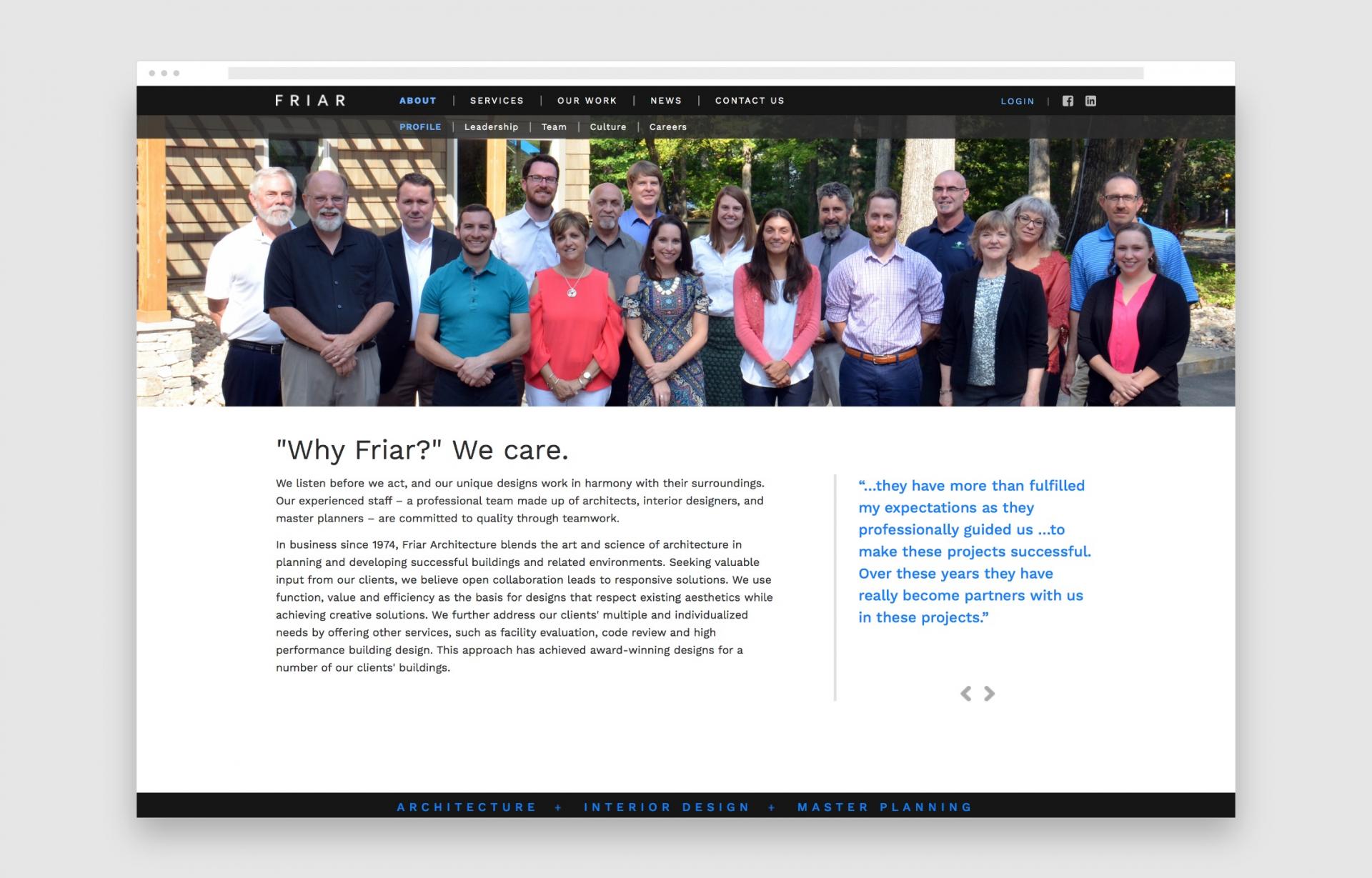This image, sourced from the Friar website, presents a comprehensive overview of the company’s offerings and team. At the top of the webpage, navigation tabs for Services, Our Work, News, Contact Us, alongside login options and social media links for Facebook and Instagram, are clearly visible. 

Under the 'About' section, further subsections include Profile, Leadership, Team, Culture, and Careers. The webpage features a diverse group of Friar team members, depicted in a professional ensemble of work attire—ranging from dresses and pant suits for women, to dress shirts, pants, and collared shirts with ties for the men.

Central to the page is the company's ethos, conveyed through the headline “Why Friar: We Care.” It highlights their commitment to attentive client service and unique, harmonious designs backed by a professional team of architects, interior designers, and master planners. Established in 1974, Friar Architectural prides itself on blending the art and science of architecture and planning, crafting distinctive buildings and environments. They emphasize open collaboration, ensuring designs are functional, valuable, efficient, and aesthetically respectful.

Friar also addresses diverse client needs with additional services such as facility evaluation, code review, and high-performance building design, earning them numerous accolades for their client projects. Adjacent to this, a testimonial in blue text praises Friar’s professionalism and partnership, highlighting their success and fulfillment of client expectations.

At the bottom of the page, more navigation tabs offer insights into Friar’s expertise in Architecture, Interior Design, and Master Planning, promising a detailed exploration of their specialized services.